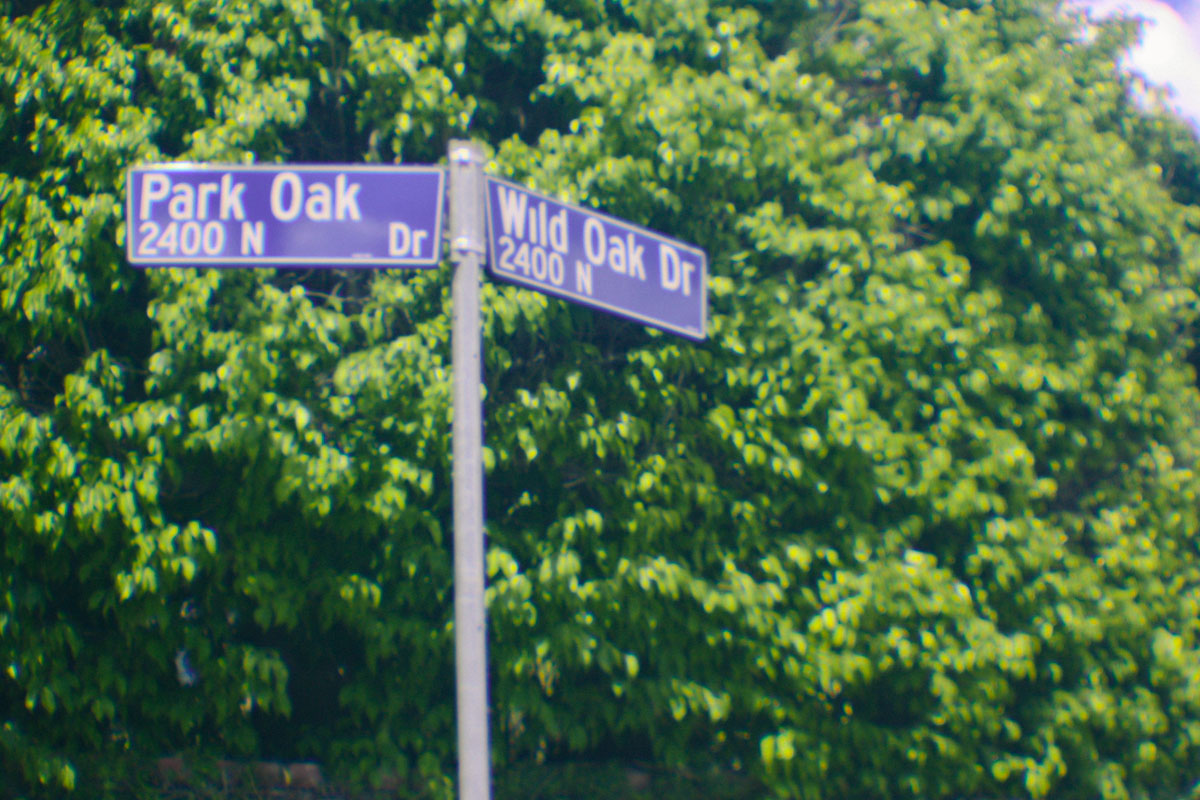The photograph captures a slightly blurry and grainy roadside scene featuring a gray metal pole with two blue signboards bordered in gray at its top. The left signboard reads "Park Oak DR 2400 N," while the right one says "Wild Oak DR 2400 N." In the background, there is a lush, green, leafy expanse that appears to be the top of a large tree or potentially a giant bush, adding a vibrant, natural element to the scene. The bottom of a building is faintly visible beneath the greenery, hinting at an urban setting softened by the plant life. The image, with its mix of nature and street signage, offers a picturesque and calming view amidst what might otherwise be a typical urban landscape.